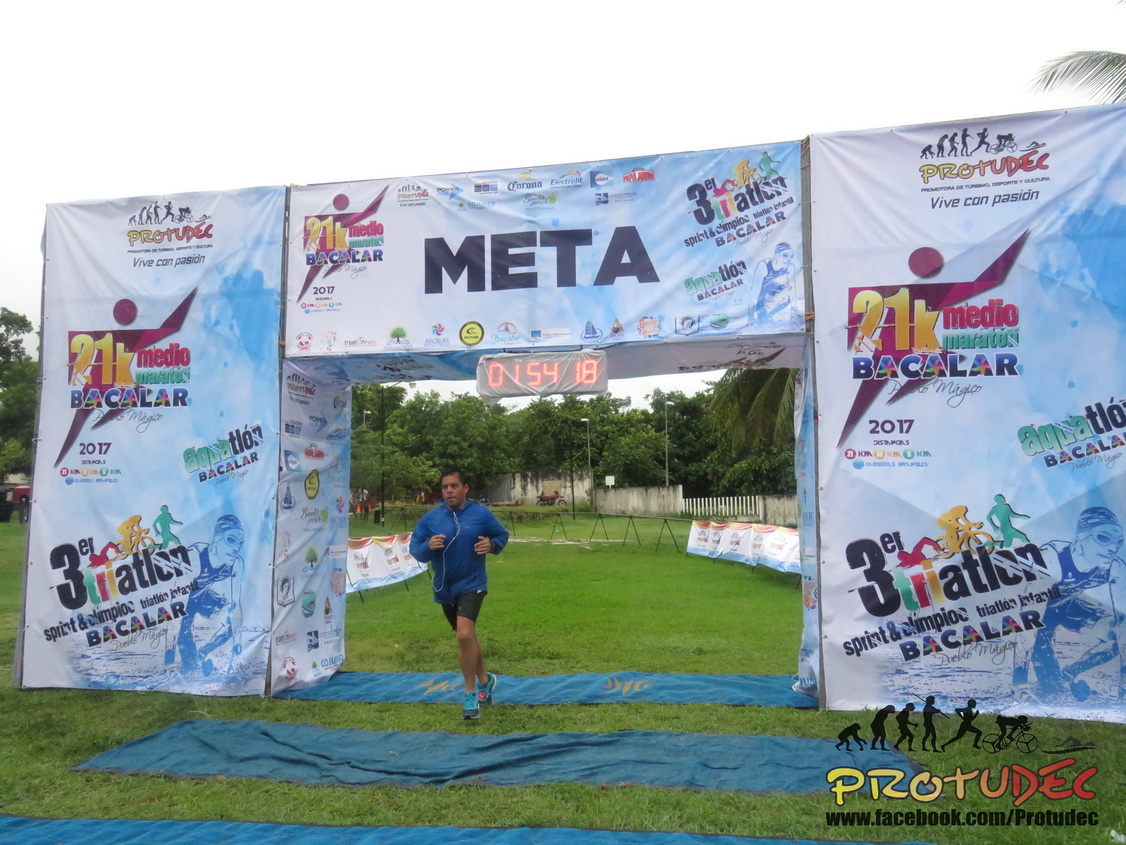In the image, a runner with dark features, dressed in a blue long-sleeve sweater and black shorts, is sprinting to the left beneath a 90-degree angled archway signifying the finish line of what appears to be a marathon or triathlon. The archway, prominently branded with "Meta" and "Pro2Deck," and adorned with blue tarps on the ground beneath, features a digital clock displaying "015418" to record race times. The structural design of the archway showcases an evolutionary motif transitioning from an ape to a swimmer, symbolizing the progression and endurance of the athletes. In the distant background, grass, fences, and a building are visible, suggesting an outdoor event setting. The bottom right corner of the image displays the Pro2Deck logo, accompanied by their web address, www.facebook.com/protudec. The event takes place under an overcast sky, with cool lighting emphasizing the energy and determination of the participants.